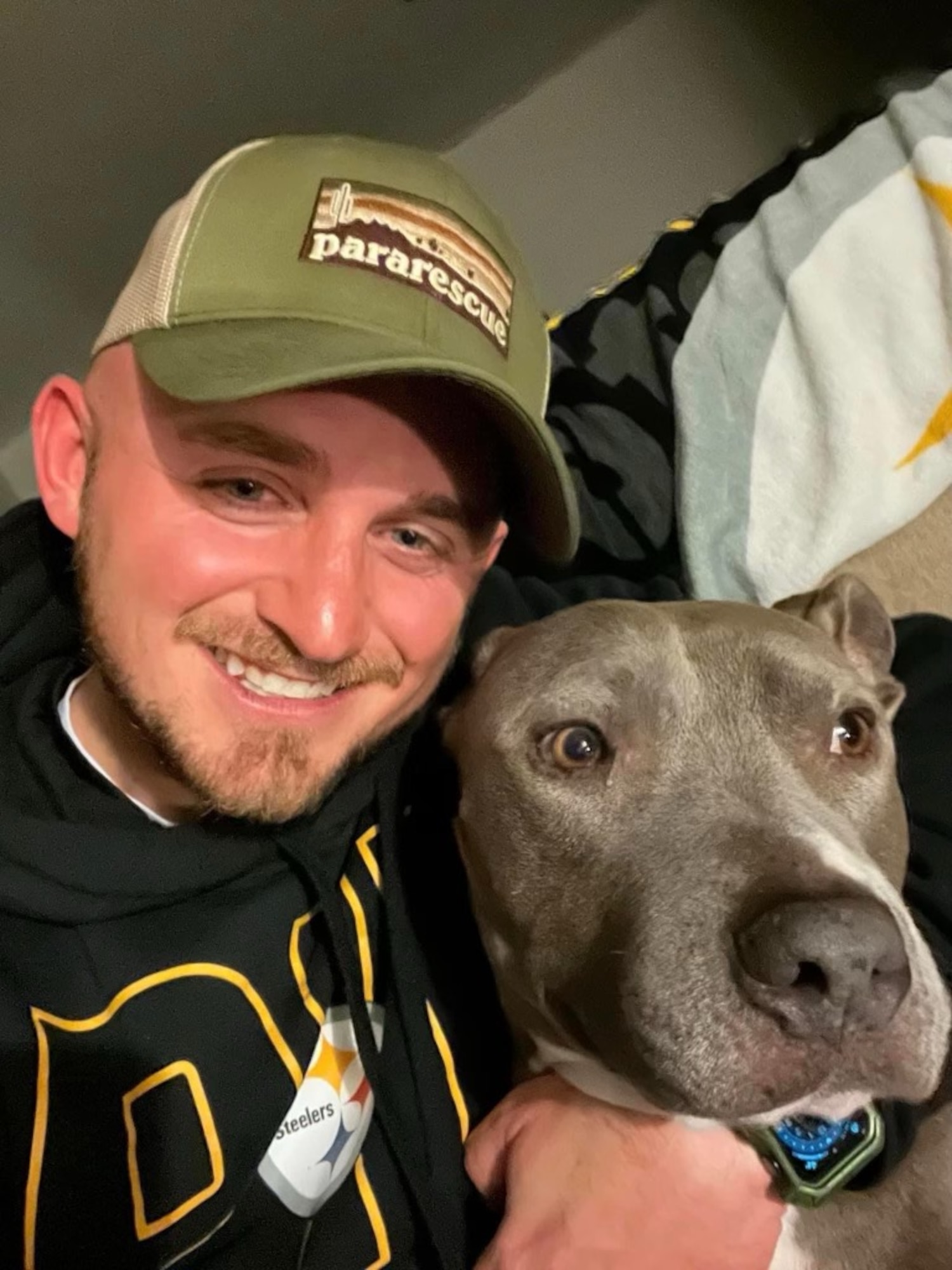In this photograph, a man and his pit bull are both facing the camera, capturing a moment of affectionate companionship. The man, situated on the left side of the frame, has his arm lovingly draped around the neck of his dog. He is smiling directly at the camera, exuding warmth and contentment, while the dog gazes off to the side, featuring a large black nose and a grayish coat. 

The man appears to be in his 30s, Caucasian, with thick brownish eyebrows, a mustache, and some stubble. He is dressed in a black sweatshirt adorned with a visible Pittsburgh Steelers logo and the word "Steelers" in bold lettering. Though partially obscured, additional letters with a gold border hint at the word "Pittsburgh."

On his head, the man wears a distinctive baseball cap that showcases a Western scene on the front panel, including a cactus and an image of the horizon. The cap is green in the front with a beige rear portion, and features the text "Para Rescue" beneath the scene.

The background is indistinct, potentially the interior of a vehicle or a room, but the close-up nature of the photograph keeps the focus squarely on the man and his canine companion.